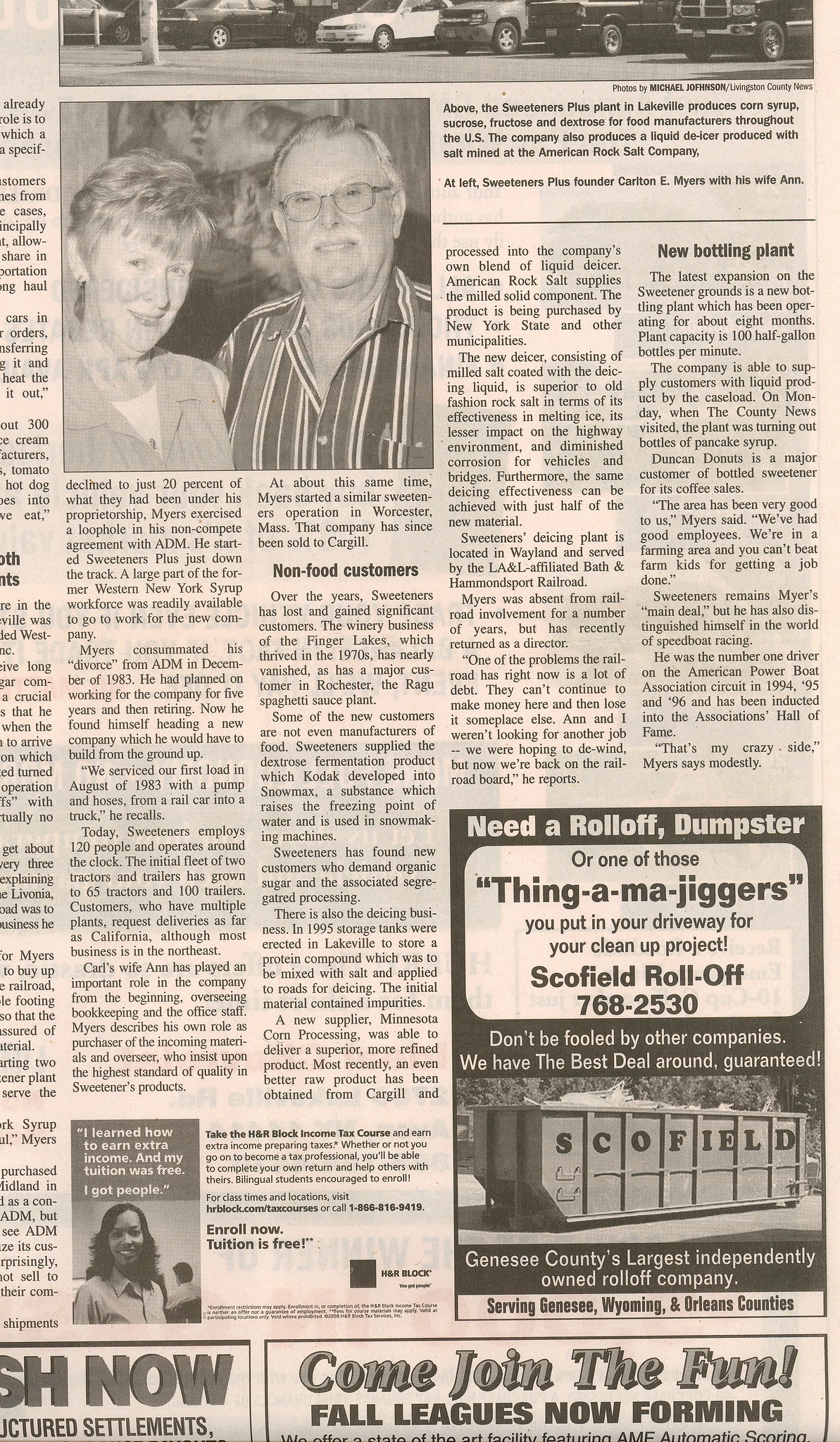The image depicts a slightly cropped page from an old newspaper, predominantly in black, white, and grayscale. The central piece of the page is an article about the Sweeteners Plus company, featuring a prominent black and white photograph of the company's founder, Carlton E. Myers, and his wife, Ann. Both are smiling warmly at the camera, and their photo spans two columns on the left side of the page. Above their image, there's another photograph partially cut off that shows a parking lot or a row of cars, with a caption stating, "Above, the Sweeteners Plus plant in Lakeville produces corn syrup, sucrose, fructose, and dextrose." Towards the bottom right corner of the page, there's an advertisement for Roloff Dumpster services, including a whimsical mention of the product as "bigger majiggers" for driveway cleanup projects. Additional advertisements are scattered at the bottom, including promotions for Thingamajiggers, Schofield, and H&R Block, with a hard-to-read invite to join a fun fall league now forming. The leftmost part of the text is slightly cropped, making some of the articles unreadable.